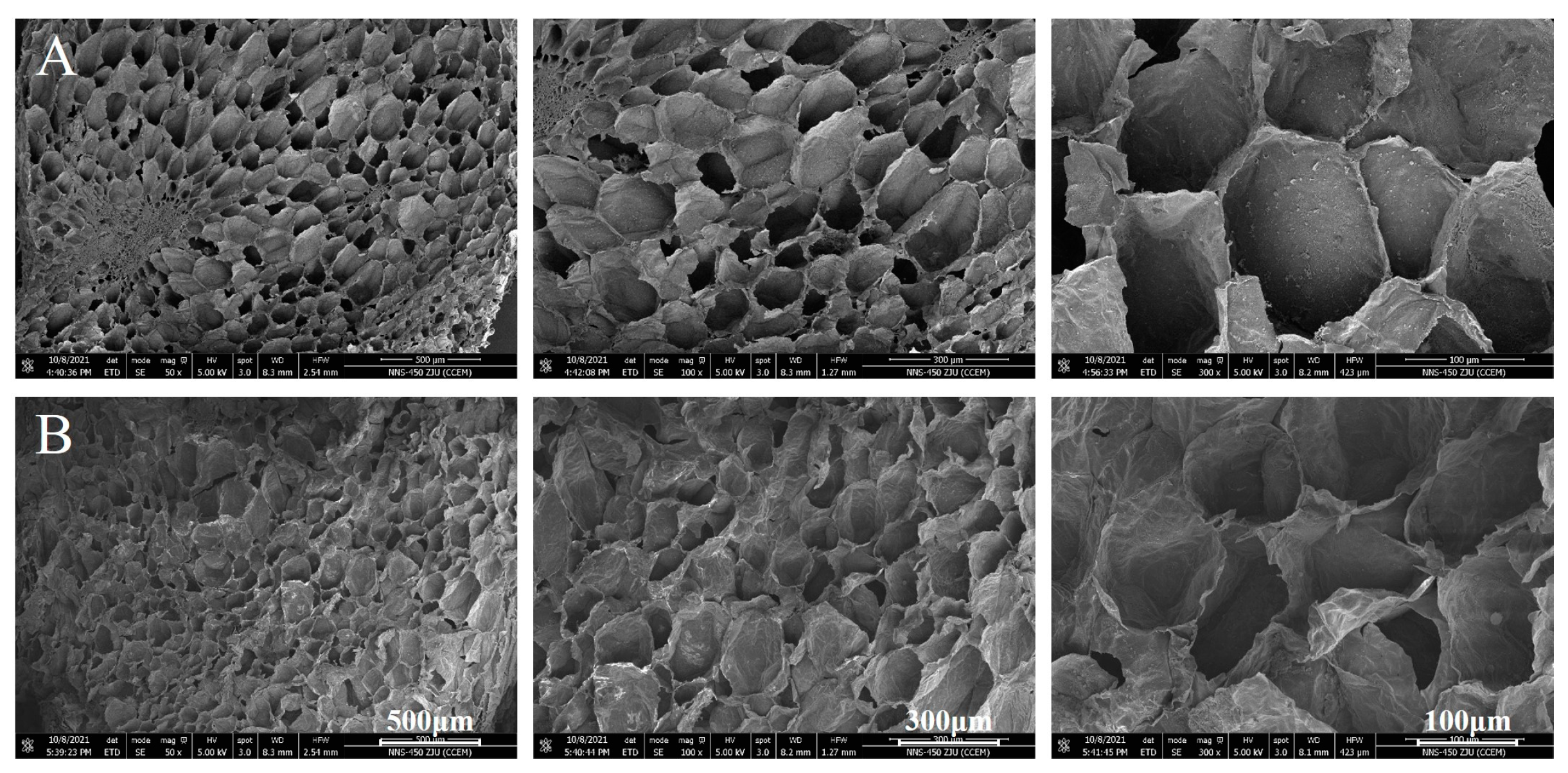The image is a wide, rectangular scientific illustration divided into two main rows, each containing three black and white microscopic close-ups, resulting in a total of six sections. The top left image is labeled "A" in white, while the bottom left image is labeled "B." Each section features various oval structures with differing magnifications, indicated by the measurements at the bottom of the rows: 500 UM on the left, 300 UM in the middle, and 100 UM on the right. Accompanying these images are detailed descriptors in small white font, including a black strip at the bottom that provides additional information such as the date "10-8-2021, 4:40:36 p.m. ETD," magnification settings like "mag 50x," and other technical details. The images display varying shades of light and dark, possibly depicting holes or caverns within the microscopic subject matter.